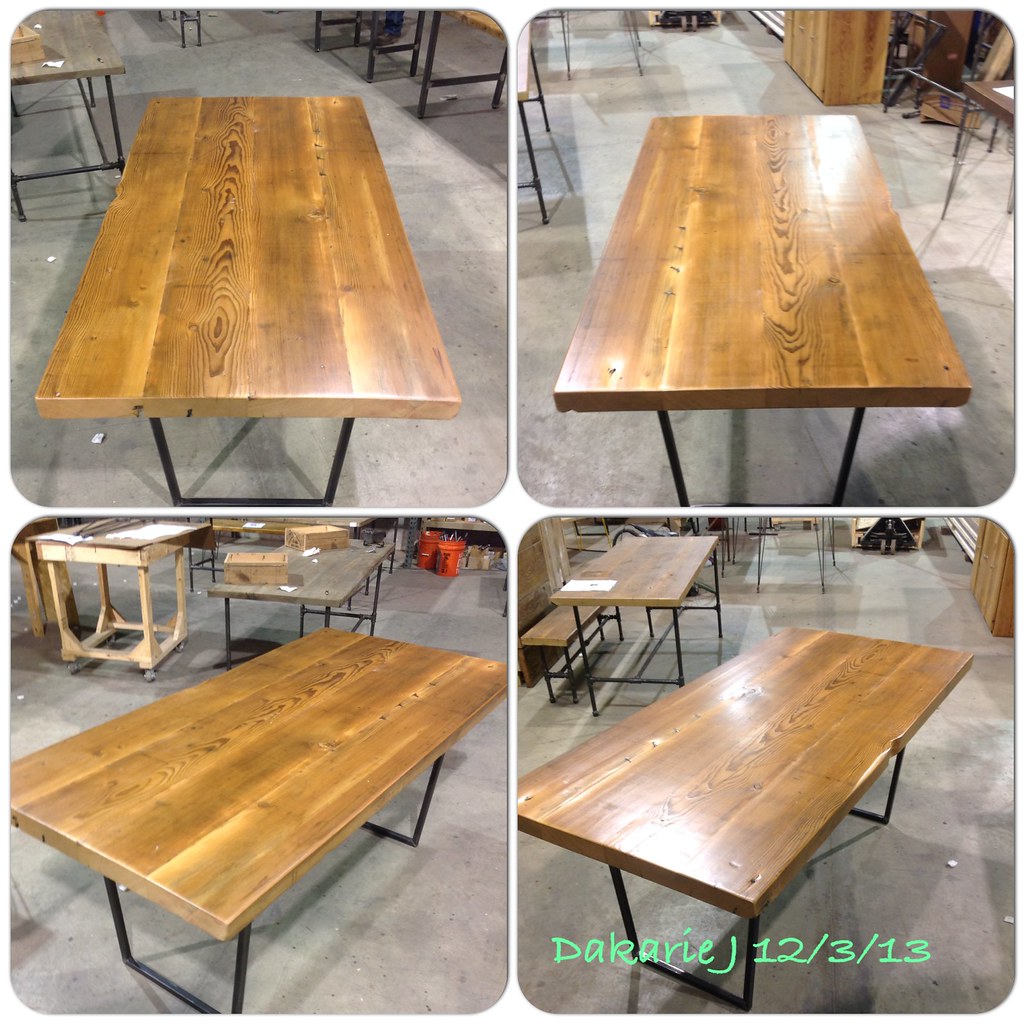The image comprises four photographs highlighting a wooden table from different angles, arranged in a 2x2 grid. The table features a medium brown wooden top with black iron legs. The top left and right photographs provide an overhead view, with the right image offering a closer look at the wood's grain and surface. The bottom left image captures the table at a slight angle, showcasing the iron legs and the wooden top's alignment. The bottom right image mirrors this angle but focuses on a noticeable imperfection—a chip in the wood on the right-hand side of the table. This photograph also includes a watermark, "DAKAREJ 12-3-13," at the bottom. The surrounding environment suggests a workshop setting, visible through various other tables and benches in the background, some with scattered sheets of paper and white debris on a concrete floor. Additionally, there are oversized orange bucket-like objects seen in the far background.